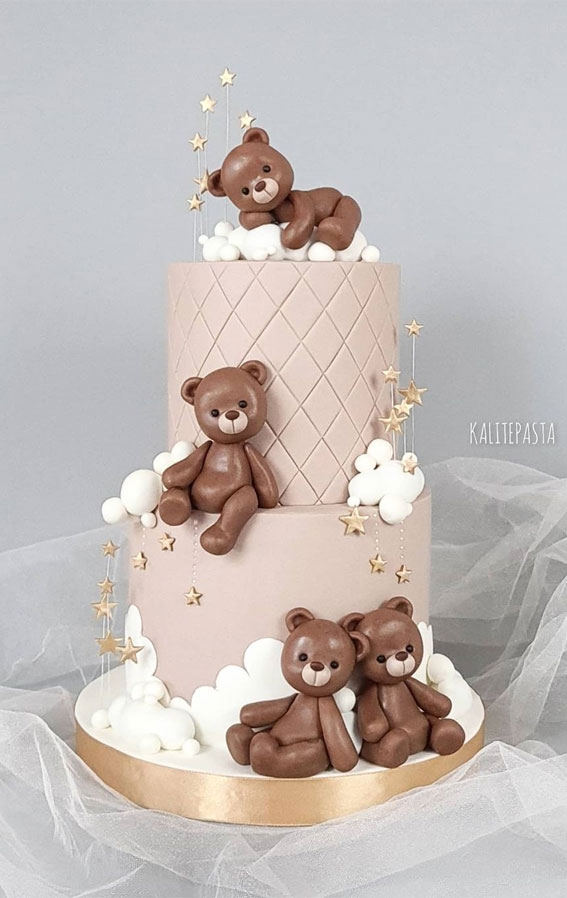The image showcases an intricately designed, three-tiered wedding cake against a grey, semi-transparent background that resembles tissue paper or tule. The cake features a smooth fondant finish and is adorned with whimsical decorations, perfect for a child's event or a themed celebration. The base tier of the cake is encircled by white fondant clouds and two teddy bears seated whimsically. The second tier continues the cloud motif, topped with stars and a single teddy bear facing forward. Rising to the top tier, a teddy bear reclines on a cloud, with stars delicately positioned above its head. The overall presentation includes fondant marshmallow balls and elements possibly made of chocolate, adding to the magical theme. The cake rests on a layer of thin white lace mesh, contributing to the delicate and ethereal aesthetic. The entire scene is signed off with a credit to "Calite Pasta," indicating the creators or inspiration behind this delightful confectionery masterpiece.